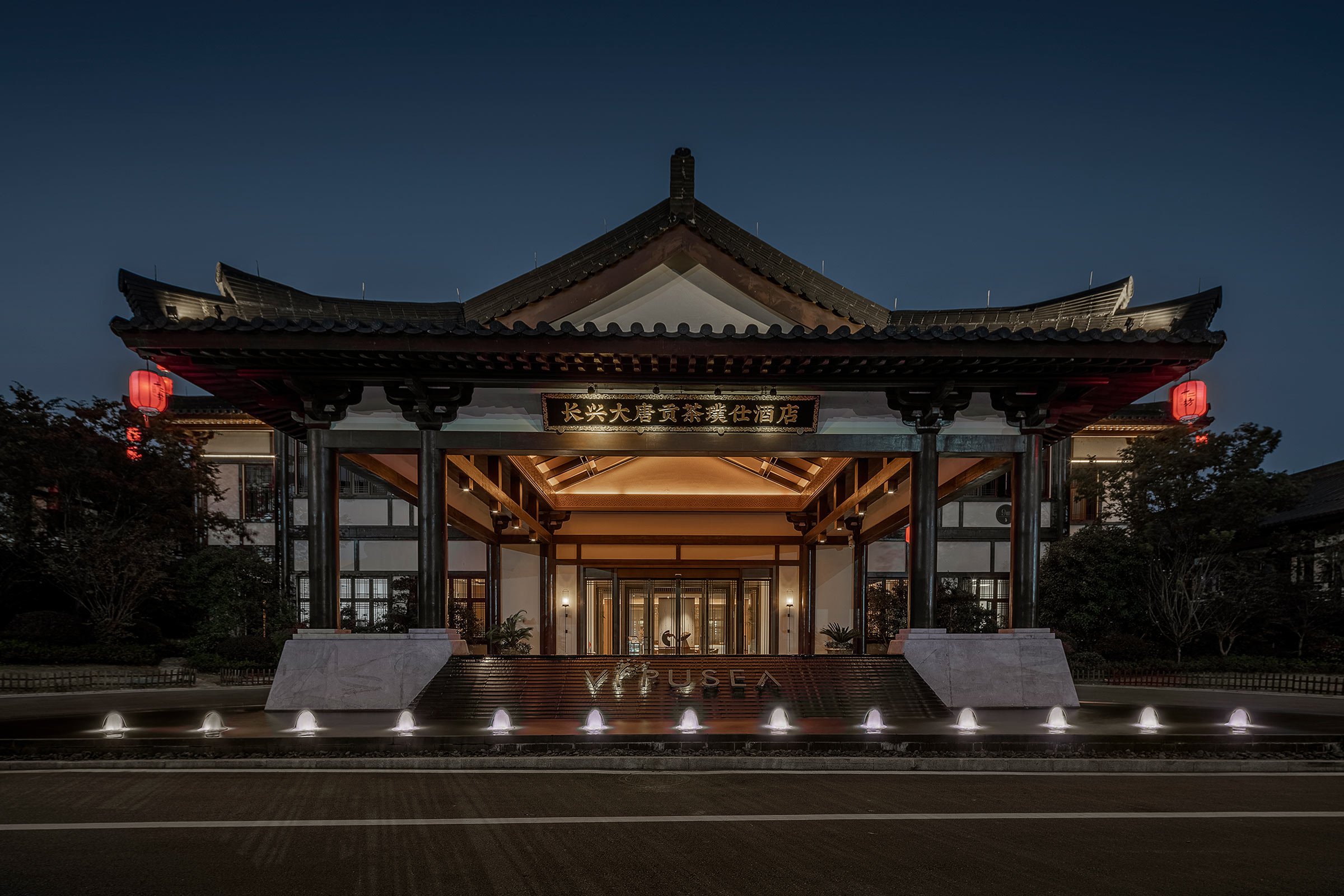This photograph, taken at night, depicts the exterior of an Asian temple, likely Japanese. The ornate wooden trim is detailed, with the corners of the temple’s roofs elegantly curved upward in the traditional Asian style, creating pointed triangular shapes. Prominent wooden pillars stand at the front of the building, supporting a high ceiling with large exposed wooden beams. A gold banner featuring Asian characters or Japanese writing hangs prominently at the top.

The temple’s façade features a line of small, white domed lights along the front, providing low illumination and highlighting the structure's intricate details. Red lanterns hang on either side of the front, adding a touch of color and traditional ambiance. The temple's color scheme primarily includes black, white, and brown hues.

Visible through the large glass doors, the interior appears spacious with a high ceiling that peaks in the center. Outside, at the street level, there is a notable water feature with numerous underwater lights and fountains, enhancing the serene and majestic atmosphere of the scene. The dim night sky forms the backdrop, devoid of people or animals, emphasizing the temple's tranquil setting. No English writing is present in the image, and the specific location remains unspecified.